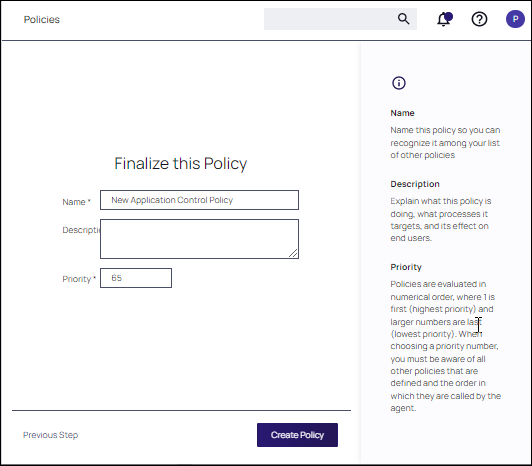This screenshot features a policy form interface. In the upper left-hand corner, the label "Policies" is displayed in black text. Adjacent to this, on the right, is a search bar, followed by an "Alerts" button marked by a purple dot. Further to the right is a "Help" link, represented by a circle containing a question mark. Next to this, there is a dark blue or purple circle with a white letter "P" inside it.

Below these elements, the main section of the form begins with a title in bold letters reading "Finalize This Policy." Directly underneath, there's a text box labeled "Name," which currently has the placeholder text "New Application Control Policy." Following this, a section titled "Description" includes an accompanying text box for further details. Beneath this, the form features a "Priority" section, highlighted with an asterisk for required input, showing the number "65" in the corresponding box.

At the bottom of the page, on the left, the words "Previous Step" are visible. Positioned to the right of this is a prominent purple button with white text that reads "Create Policy."